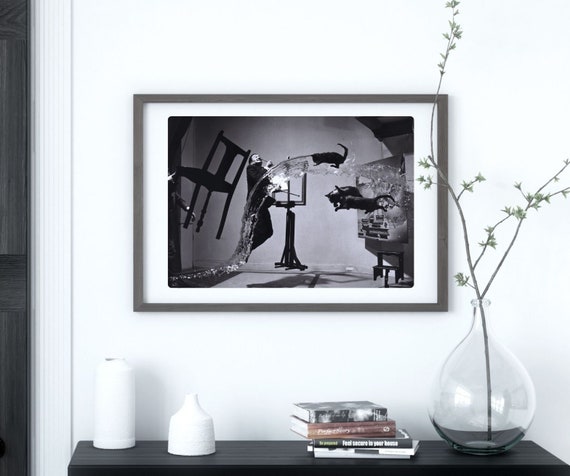The photograph captures a painting that is prominently displayed on a white wall inside a room, possibly near the end of the room as suggested by a doorway visible to the left. The artwork, encased in a dirty green or greenish-brown frame, depicts a surreal and whimsical scene in black and white. Central to the painting is a man, presumably a wizard, who is floating along with several other elements: a chair, a curved stream of water, an easel, and three black cats. The man, who has a peculiar smile, holds an undisclosed object in his hand, and there is a smaller floating painting on the right-hand side within the larger painting.

Beneath this artwork is a wooden table with a smooth surface. On the table, slightly off-center to the middle, are four or five stacked books, among which one is distinctly red, popping out against the monochrome setting. To the right, there is a clear glass vase containing a branch with sprouting green buds. On the left side of the table, there are two white objects - likely candles or implements possibly associated with incense, contributing to the room's aesthetically cohesive corner.